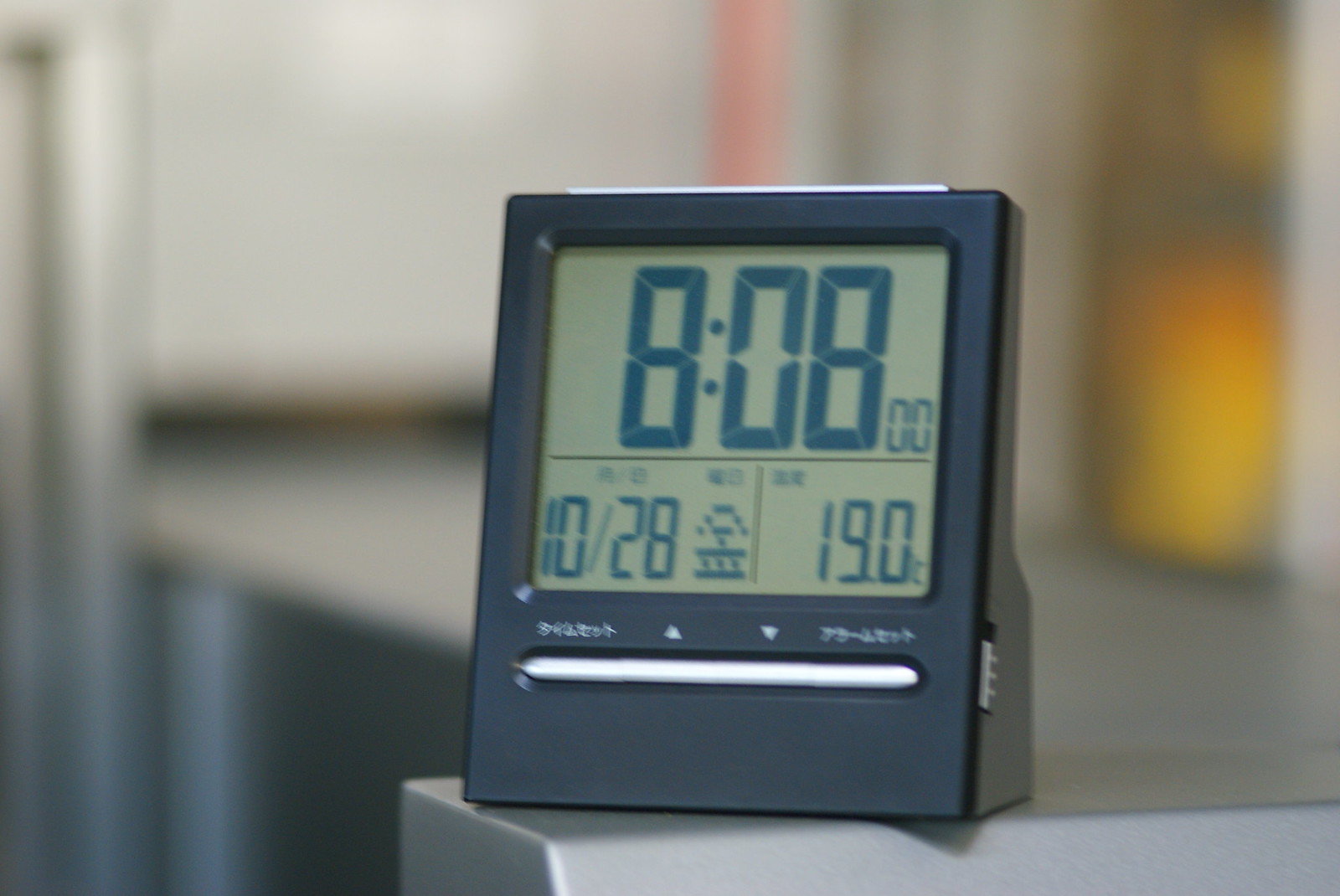This photo features a small, portable digital clock encased in black plastic. The clock, which stands a couple of inches in height, has a digital screen with a greenish-gray background displaying black digital numbers. The time shown on the screen is 8:08, the date is October 28th (10/28), and the temperature is set to 19 degrees Celsius. Additional elements include Japanese text and control arrows on the top left and right of the screen. While a silver bar or big button is present at the bottom of the clock, it appears somewhat blurry. The clock is placed on the corner of a metal surface in a blurry background that includes vertical poles and yellow lights.